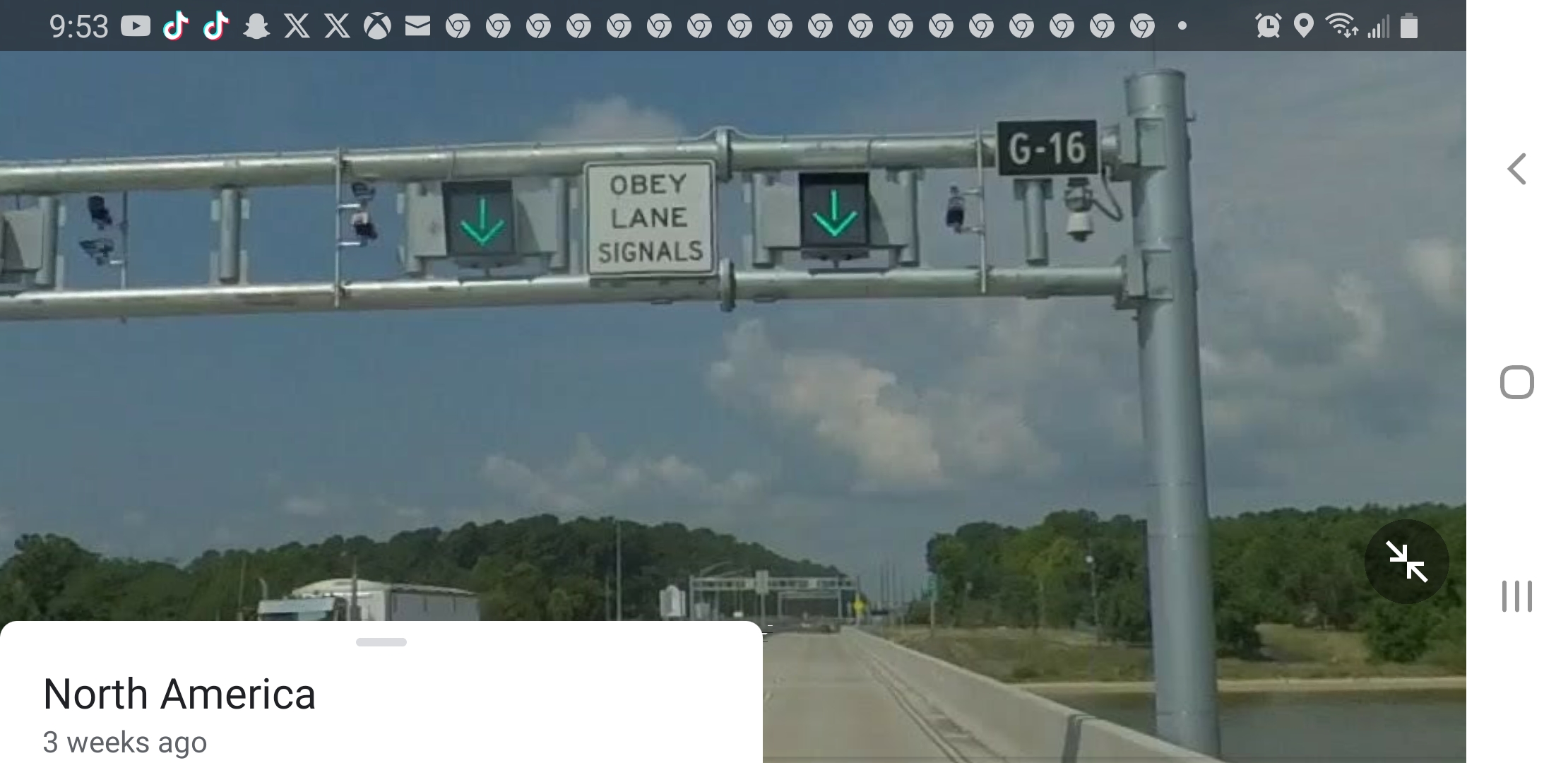**Caption:**

The image appears to be a screenshot taken on a phone of an outdoor scene. At the top of the screenshot, there is a black bar with white icons and text. Starting from the left, it displays the time as "9:53". Next, there is a YouTube play button, followed by two TikTok icons, the Snapchat logo, and two Twitter icons represented by an "X". Then, there is the Xbox symbol, characterized by a circle with a clear "X" through it, followed by an envelope icon indicating email.

Below this top bar, a significant portion of the screen is occupied by a massive numerical sequence which starts at 1 and goes all the way up to 77, with certain numbers repeating multiple times throughout the sequence.

In the bottom left corner of the image, there is a white rectangle. On the right-hand side of the screenshot, the word "North America" is displayed in black text. Below this, in a lighter gray text, it reads "3 weeks ago."